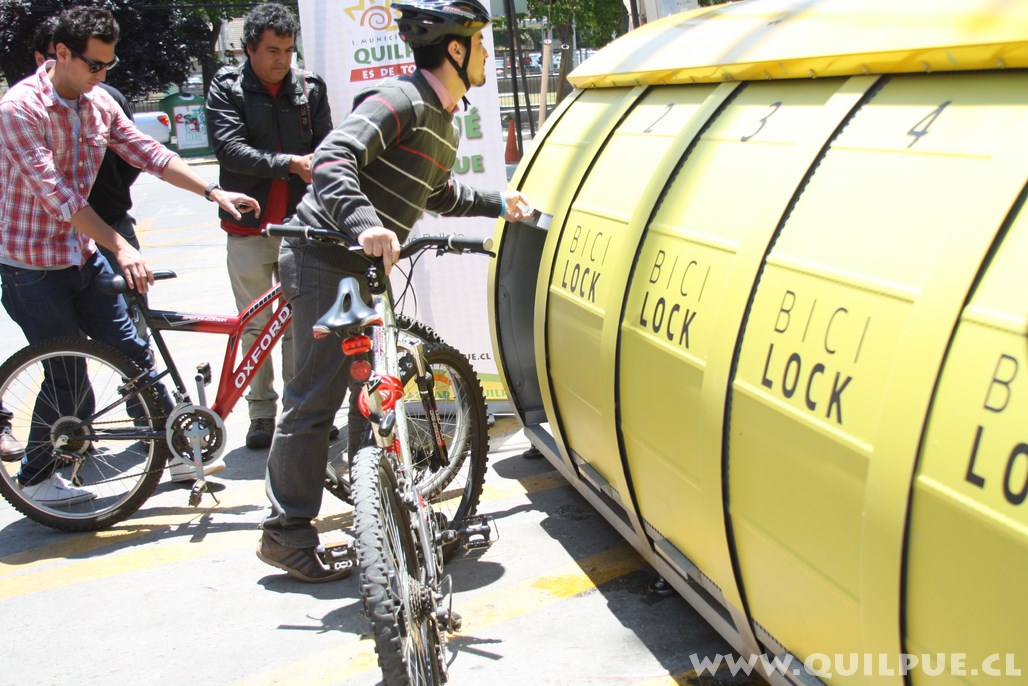In this outdoor daytime photograph, a rectangular image that is wider than it is tall, three men are gathered on the left side, each with mountain bikes featuring thick tires. One man is actively opening a door of a large, cylindrical yellow container on the far left, marked with "B-I-C-I lock" and numbered 2, 3, and 4, indicating compartments for securely storing bicycles to protect them from theft. The opaque gray watermark "www.quilpe.cl" is visible in the lower right-hand corner. The container doors can be lifted to allow bike storage, and the ground next to the cylindrical lock area consists of black pavement with diagonal yellow stripes. The background reveals a park landscape with green trees, a white sign, a street with a truck, traffic cones, and additional elements like a trash can, indicating a typical urban park setting.